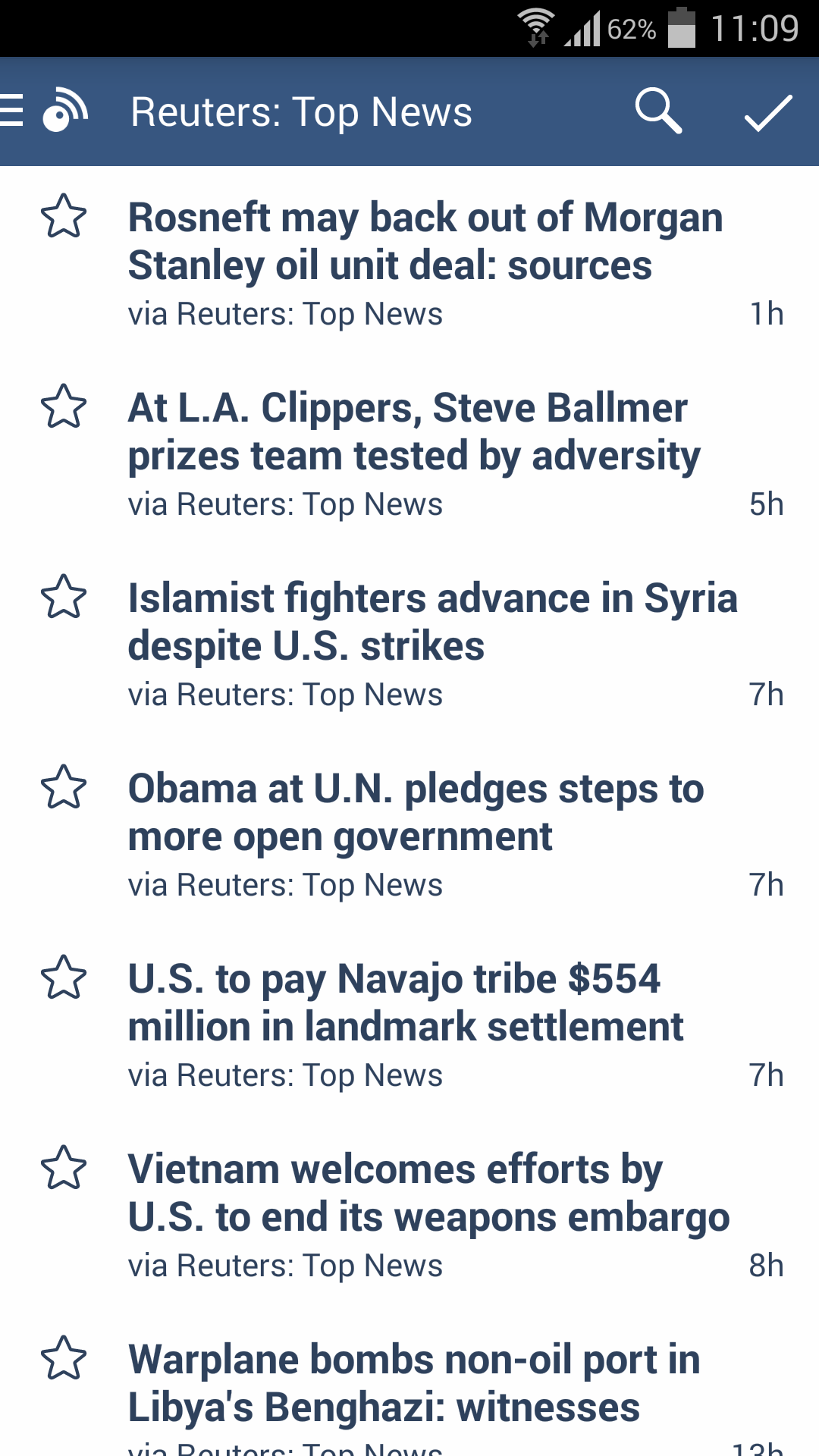This screenshot from an Android phone displays the home screen of the Reuters app under the "Top News" section. Key details visible include:

- **Wi-Fi and Cellular Data Status**: Both are connected.
- **Battery Level**: 62%.
- **Time**: 11:09 AM.

The app interface shows a search bar at the top, alongside a check mark icon. The headlines of the top news articles and their respective posting times are listed as follows:

1. **"Ross Neft may back out of Morgan Stanley oil unit deal sources"** - 1 hour ago
2. **"At LA Clippers, Steve Ballmer prizes team tested by adversity"** - 5 hours ago
3. **"Islamist fighters advance in Syria despite US strikes"** - 7 hours ago
4. **"Obama at UN pledges steps to more open government"** - 8 hours ago
5. **"US to pay Navajo tribe 554 million in landmark settlement"** - 13 hours ago
6. **"Vietnam welcomes efforts by US to end its weapons embargo"** - Time not specified
7. **"Warplane bombs non-oil port in Libya's Benghazi, witnesses"** - Title partly cut off due to screen limitation

Users have the option to mark articles as favorites using a star icon adjacent to each headline.